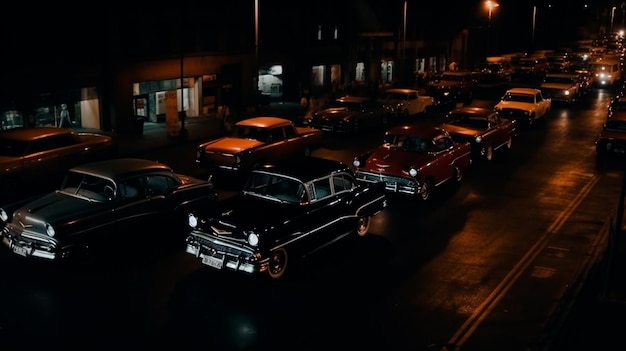The photograph captures a striking nighttime scene featuring a long line of vintage cars from the 1940s to the 1960s, all illuminated by their headlights. The street is populated with shiny old cars, predominantly in shades of black, maroon, gray, and red. The scene unfolds under dim, yellow streetlights, with two discernible rows of cars stretching deep into the frame.

To the left, illuminated buildings with businesses line the sidewalk, though specific details are hard to distinguish due to the darkness. There are some painted lines visible on the pavement, adding to the nostalgic atmosphere. Despite the limited lighting and clarity, the image centers unmistakably on this seemingly endless, orderly procession of classic automobiles driving through the night.